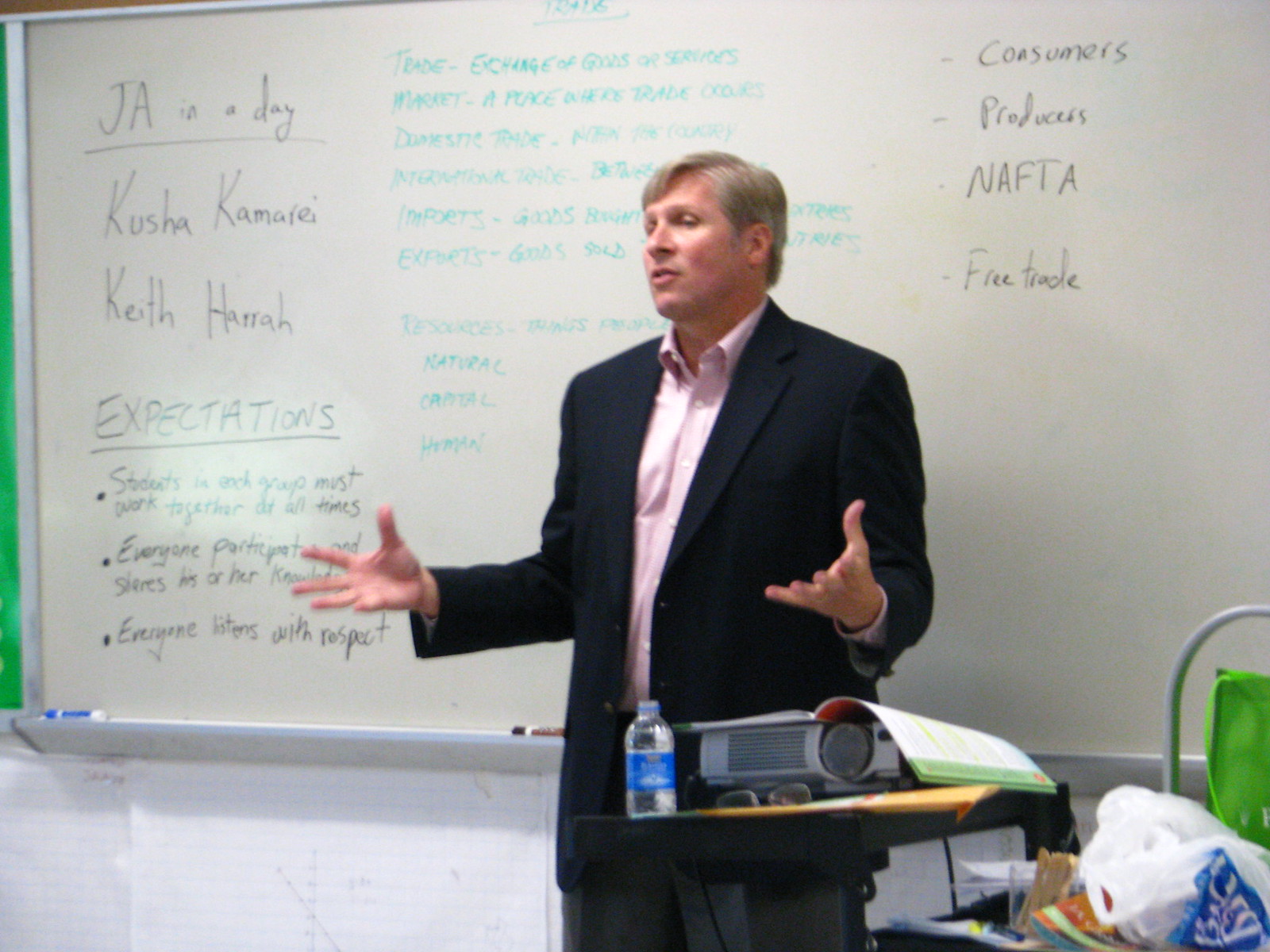A man, presumably a teacher or presenter, stands in front of a large, wall-spanning whiteboard, explaining concepts to a class. Clad in a black suit jacket and a light blue button-down shirt, he gestures animatedly with both hands raised. His light brown, graying hair adds a distinguished touch to his appearance. In front of him, a small cart table holds a projector, his glasses, a booklet, and a bottle of water, from which he likely refers to while teaching. The expansive whiteboard behind him, which dominates the backdrop except for the visible wall section below his waistline, is filled with a plethora of information. There are three columns of text: the center comprises detailed teaching points in bright green marker, while the left and right columns, written in black, include labeled sections such as "J.A. in a Day" with names Kusha Kumari and Keith Hara, and terms like "Consumers," "Producers," "NAFTA," and "Free Trade." The board is meticulously organized with headings, bullet points, and underlined topics like "Expectations," signifying an economics-related lesson. The setting is one of active instruction, with the man clearly engaging his audience through both verbal and non-verbal communication.